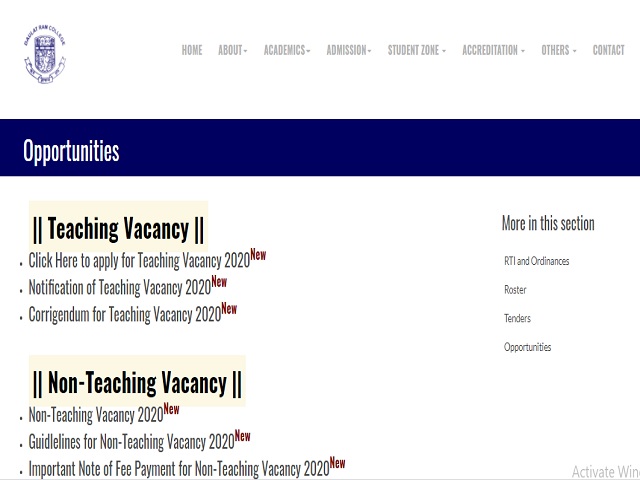The image showcases a detailed layout of a website.

**Top Section:**
- In the top-left corner, there is a dark blue logo featuring text at the top, a curved line at the bottom, and a shield-shaped emblem in the center.
- To the right of the logo, there is a navigation bar with eight categories in gray text on a white background: Home, About, Academics, Admission, Student Zone, Accreditation, Others, and Contact.

**Middle Section:**
- Below the navigation bar, there is a dark blue banner with "Opportunities" written in white text.

**Opportunities Section:**
- This section is divided into two categories: Teaching Vacancy and Non-Teaching Vacancy.
- Under "Teaching Vacancy," there are three options:
  - "Click here to apply for Teaching Vacancy 2020"
  - "Notification of Teaching Vacancy 2020"
  - "Core Agendum for Teaching Vacancy 2020"
- Under "Non-Teaching Vacancy," there are three options:
  - "Guidelines for Non-Teaching Vacancy 2020"
  - "Important Note of Fee Payment for Non-Teaching Vacancy 2020"
- Each of these six options is marked with a dark red "New" label to the right.

**Right Sidebar:**
- On the right-hand side of the page, there is a section labeled "More in this section" with four categories listed below:
  - RTI and Ordinances
  - Roster
  - Tenders
  - Opportunities
- At the very bottom right corner, the section is labeled "Activate When."

This detailed description provides a comprehensive visualization of the website layout, guiding users to relevant sections and categories efficiently.